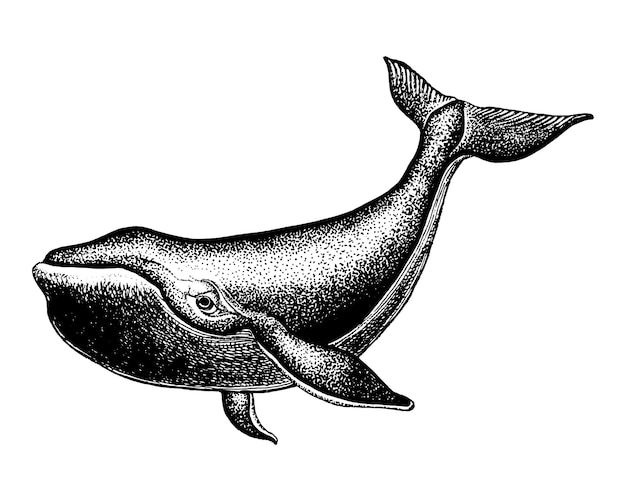This image depicts a highly detailed black-and-white line drawing of a mature humpback whale in a three-quarter view position. The whale's head is oriented to the left while its tail curls up toward the upper right corner of the image. The drawing captures the left eye and includes the full left fin and a part of the right fin under its belly. The whale's body, detailed with a series of white spots and stripes, displays a mix of shades: dark along the top with lighter tones on the belly and scattered black dots. The mouth is closed, marked by a slight hump on top, and its pupil is distinctly black. The tip of the tail showcases long white stripes, and the entire aquatic scene is set against a plain white background, focusing solely on the whale's intricate and elegant form without any additional elements.